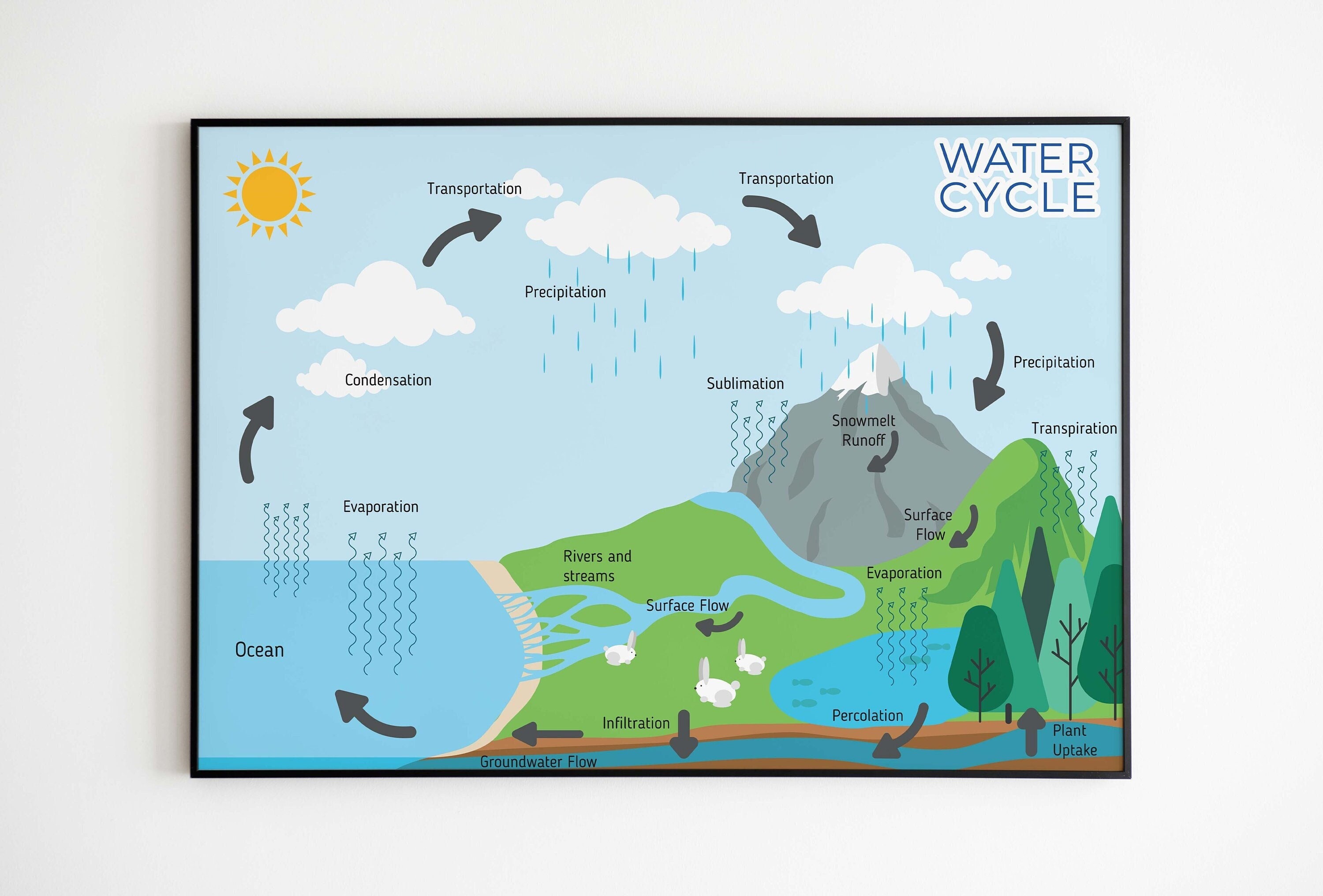The image showcases a detailed illustration of the water cycle, captured as a photograph of a framed print hanging on a plain white wall. The painting, encased in a black frame, features a light blue background and vector-based imagery without black line art. In the top left corner, a sun shines down on the scene, while "Water Cycle" is written in black letters with a white outline in the top right corner.

The illustration meticulously depicts the stages of the water cycle. Starting from the ocean on the left, it transitions into land with mountains, forests, and a lake. Black arrows guide the viewer clockwise through the cycle, depicting processes such as evaporation from the lake, condensation forming clouds, precipitation as rain and snow, and water flow through rivers and underground streams.

Key details include water evaporating from the ocean, condensing into clouds, being transported and falling as precipitation onto the mountains. The rain then travels through rivers and groundwater, eventually returning to the ocean, completing the cycle. Additional noted processes are plant uptake of water and percolation into underground water flow, all contributing to the continuous loop of the water cycle.